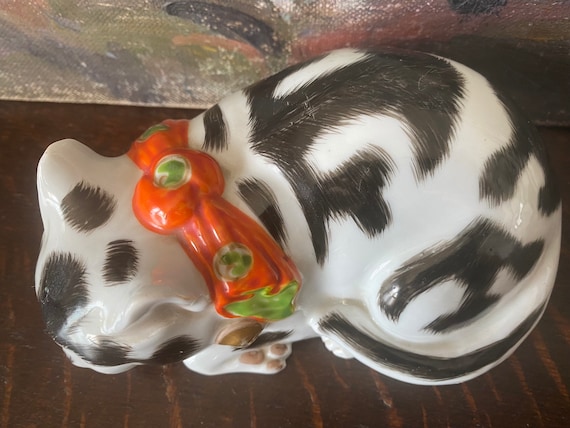This image features a close-up, top-down view of a smooth, shiny figurine that resembles a cat, likely made of glass, porcelain, or some ceramic material. The figurine is predominantly white with black patches distributed across its body and a prominently curled tail. Notably, the cat has pink pads visible on one of its paws, suggesting a meticulous level of detail. The figurine is adorned with a colorful ribbon or collar around its neck—red in color with green and white accents, almost like intricate jello-like markings or polka dots. This detailed piece sits on a light brown wooden surface, which has noticeable streaks and lines. The background also features a partly visible multicolored painting or wall with an array of colors including black, green, red, and white in a scattered, splattered pattern, adding an abstract element to the scene.